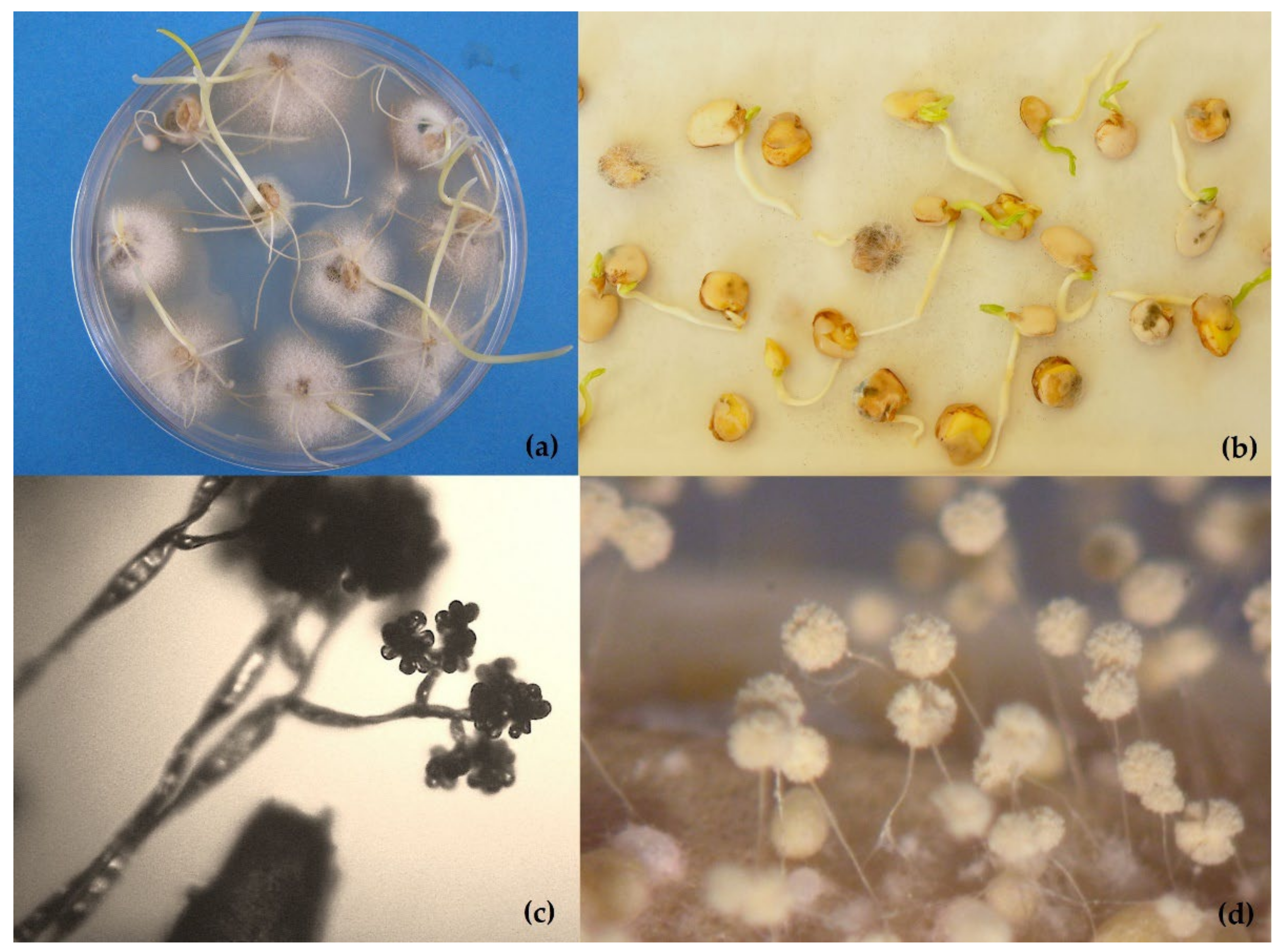The image consists of four rectangular panels labeled A through D, each showcasing various stages of germination or microscopic growth. Panel A, situated in the upper left, features a blue background with a clear plastic Petri dish containing multiple whitish seeds. These seeds exhibit greenish sprouts and roots, indicating early germination. Panel B, in the upper right, presents a creamy yellow background with rounded seeds that have burst open, revealing greenish sprouts and developing roots. Moving to panel C in the bottom left, against a similarly colored, cream background, there is a shadowy, black-and-white image resembling DNA strands branching out like miniature trees or tiny clusters. Lastly, panel D in the lower right shows a brownish background with slender, thread-like stalks ending in small, white, cotton-like puffs, each reminiscent of a microscopic field of cotton flowers. Together, these panels depict various stages of growth and microscopic structures in a detailed, scientific manner.